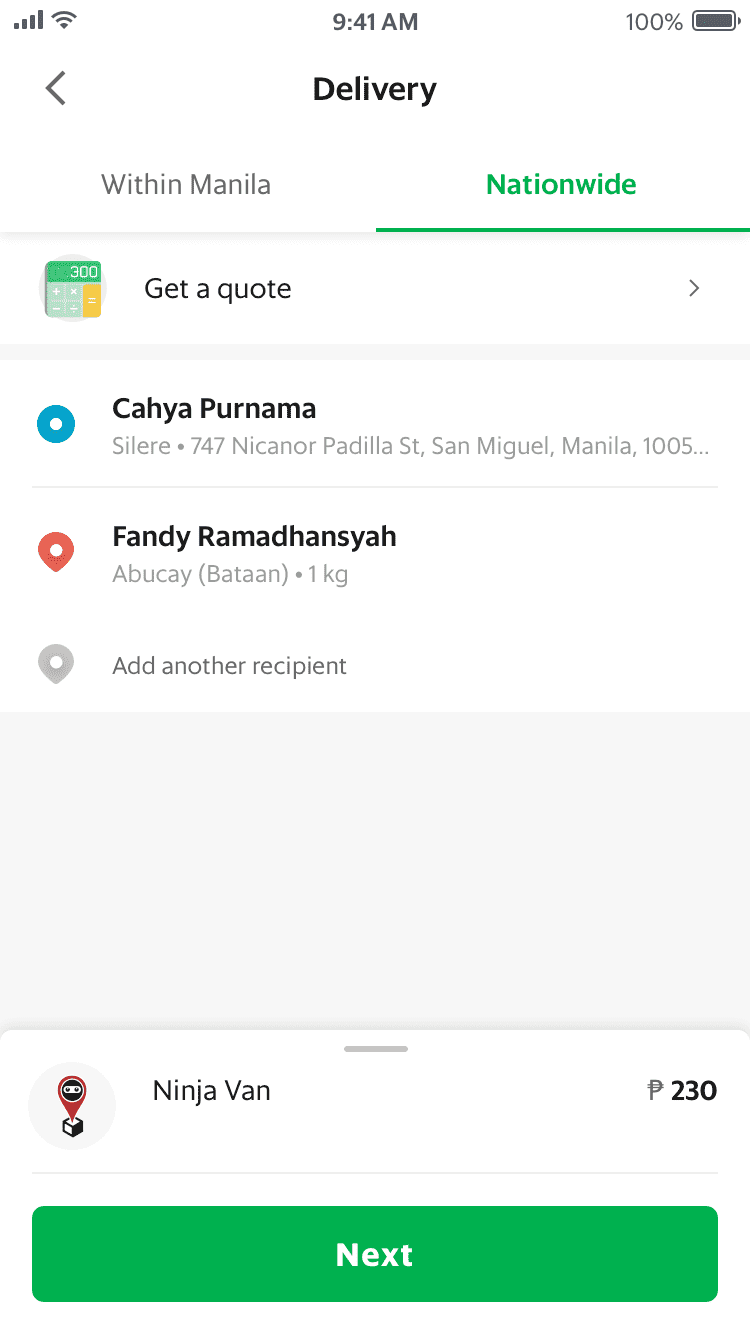This image is a cell phone screenshot depicting a delivery status page. At the very top, situated below the time, the word "Delivery" is center-aligned. To the left of "Delivery" is a back arrow icon. Below the title, there are two tabs: one labeled "Manila" in black font, and the other labeled "Nationwide" in green font with a green underline indicating it is the selected tab.

Immediately below the tabs are four information lines. The first line reads "Get a Quote" in black font accompanied by a cartoon-style calculator icon to its right. The second line contains the name "CAHYA PURNAMA" in all caps with the middle initial "S" in gray font beneath it. The address "Solaire 747 NICANOR Padilla Street, Manila" is listed below the name.

The third line presents another name, "Fandy R.", with the last name starting with "R." Finally, the fourth line indicates the weight "one kilogram" under the aforementioned names and addresses.